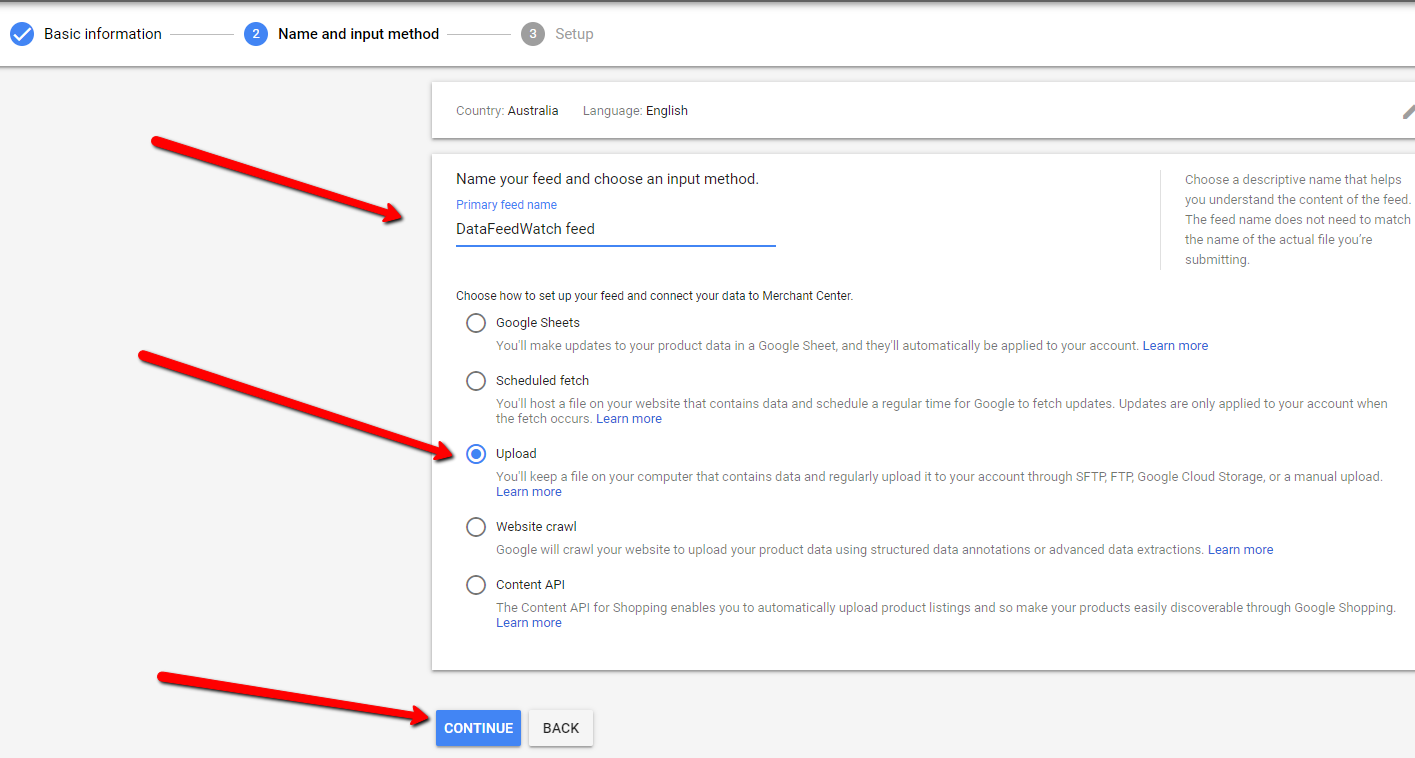The image depicts a screenshot from a form on a website, designed for user input. The interface is light-colored and features three large red arrows that have been added to guide users through the form. 

At the top of the form, there is a sequential navigation bar indicating the steps the user has already completed. Each completed step is marked with a blue circle containing a white check mark. The current position is on the second step, labeled "Name and Input Method."

Below the navigation bar, the form displays a section that reads "Country" and "Language," with "Australia" and "English" selected respectively. Following this, a larger section is presented, where two of the red arrows are pointing.

The first red arrow highlights the field labeled "Primary Feed Name," where the user has entered "DataFeedWatch Feed." This entry demonstrates the format required for naming the feed.

The second red arrow points to the "Input Method" section, where the user can select from multiple options. Each option is accompanied by a circle indicating its selection status. The "Upload" option is chosen, marked with a blue dot.

Finally, the third red arrow directs attention to the "Continue" button located at the bottom of the screen, signaling the next step for the user to proceed in the form.